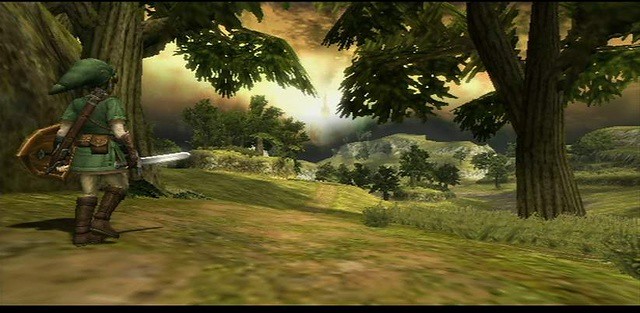In this animated scene from a video game, the central character is viewed from behind, showcasing their green hat and brown armor. They are also wearing brown boots and appear to be carrying either a knife or a shield. The character strongly resembles Zelda, standing in an expansive natural environment filled with lush greenery and numerous trees. Rolling hills and large mountains dot the landscape, suggesting vast areas to explore. The setting sun bathes the scene in a warm light, further emphasizing the tranquil, open-space ambiance. Despite the detailed environment, no other characters are present, highlighting the lone adventurer's journey through this vibrant, modern-rendered forest.